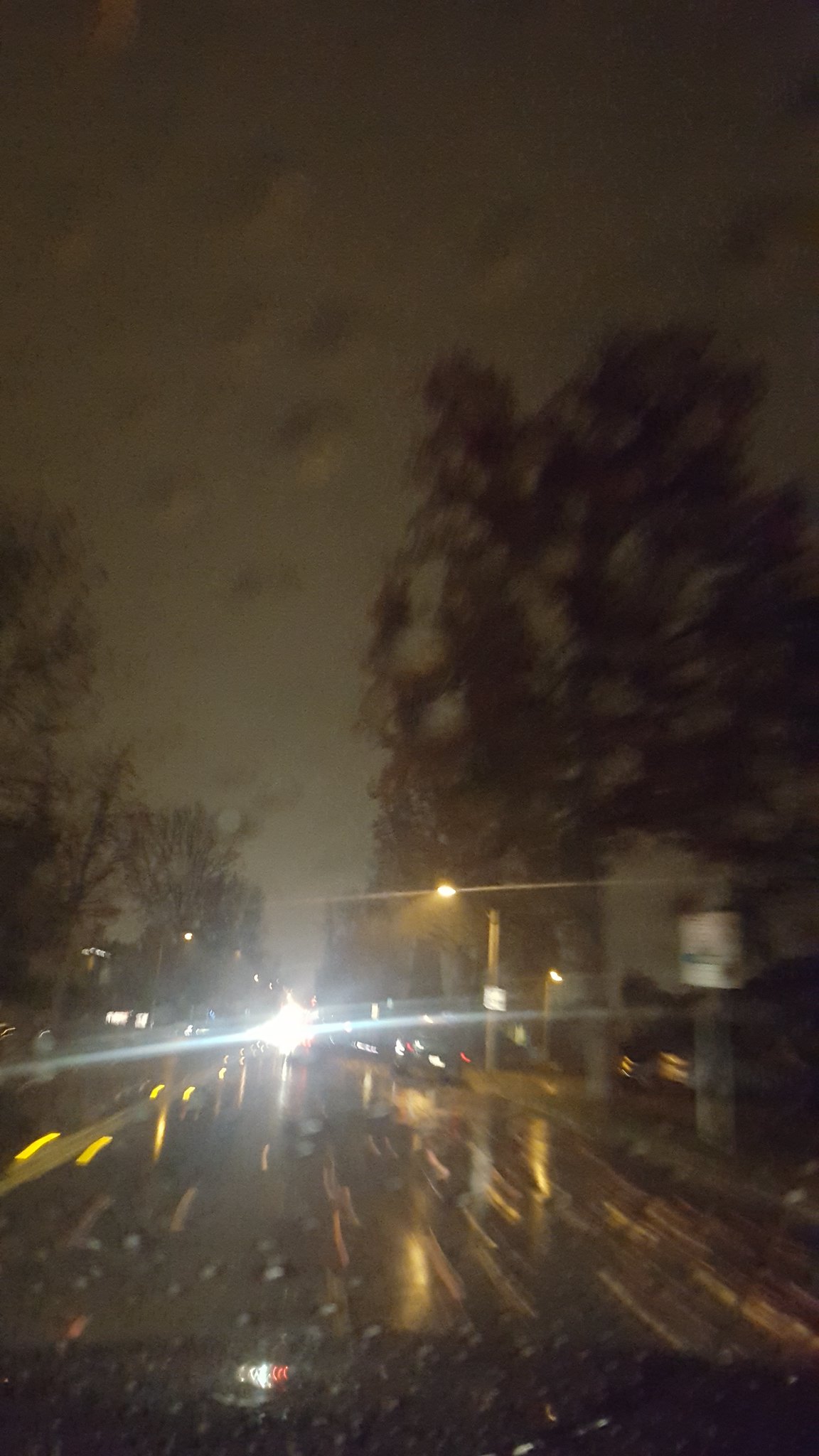This nighttime photograph, taken from inside a car, captures a rain-soaked scene through a windshield speckled with water droplets. The image is blurry, enhancing the moody atmosphere of the wet night. A glaringly bright headlight from an oncoming vehicle pierces the darkness from down the road, obscuring the vehicle itself. To the right of the road, there's a barely discernible street sign, blurred by motion and the raindrops. Tall, prominent trees flank both sides of the road, with a particularly large one on the left accompanied by smaller trees, while a bigger tree stands on the right. The sky above shows a mix of dark and lighter patches, possibly illuminated by city light pollution, reflecting the rain on the windshield. The hood of the car and some streetlights can be faintly seen through the raindrops, adding depth to the scene.